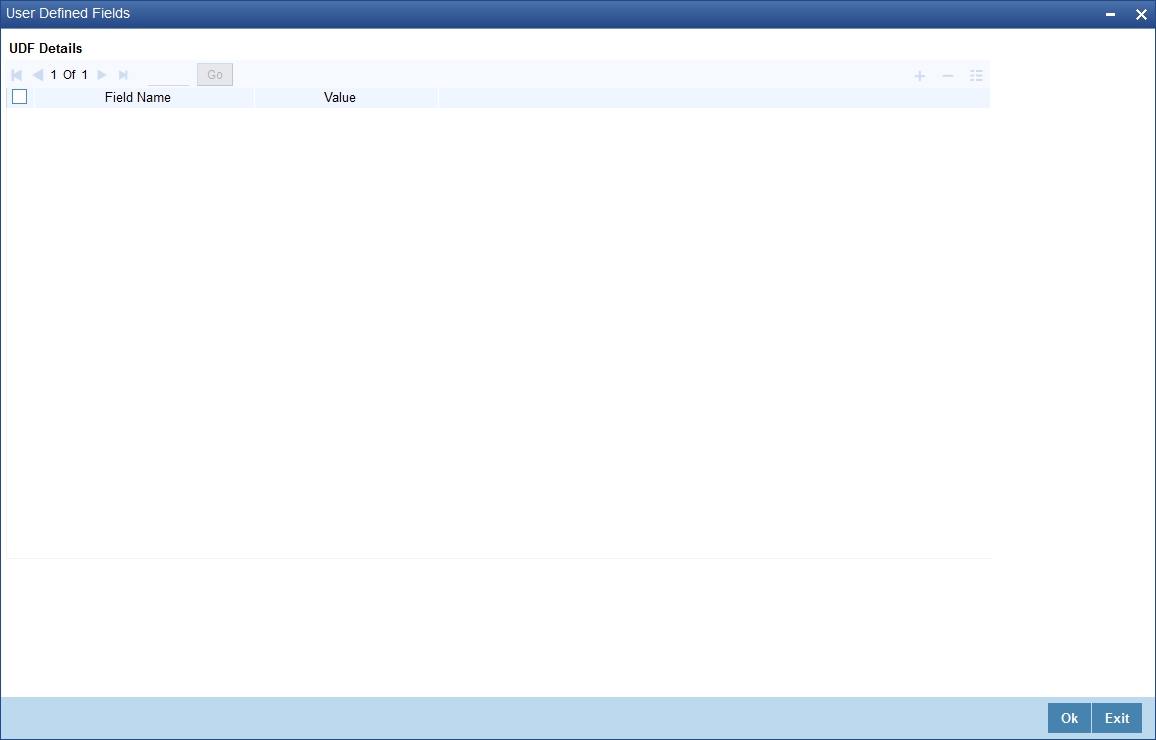### Caption

The image is a screen capture showcasing a user interface that is characterized by its simplicity and absence of data input. At the top-left corner, it is labeled "User Defined Fields," with the minimize and close icons positioned to the right. Below this heading, the section titled "UDF Details" appears in black text.

Immediately beneath, there is a blue horizontal rectangle featuring a navigation toolbar. This toolbar includes several buttons: a 'Repeat' button, a left-facing arrow, a "One of One" indicator, a right-facing arrow, and a 'Fast-Forward' button. Next to these, there is a field labeled "Go."

The central area of the screen is predominantly occupied by a large, empty white space, designated for data entry yet currently unused. A single checkbox titled "Field Name" along with an adjacent "Value" field is located just below the "Go" field.

At the bottom, the interface displays a light blue horizontal rectangle, with two dark blue buttons—marked "OK" and "Exit" in white font—situated in the bottom-right corner. The overall aesthetic of the interface evokes the look and feel of the older Windows 98 operating system, particularly in terms of font and layout design. 

The image clearly indicates that the "User Defined Fields" section has been opened, although no specific data has been entered into it.